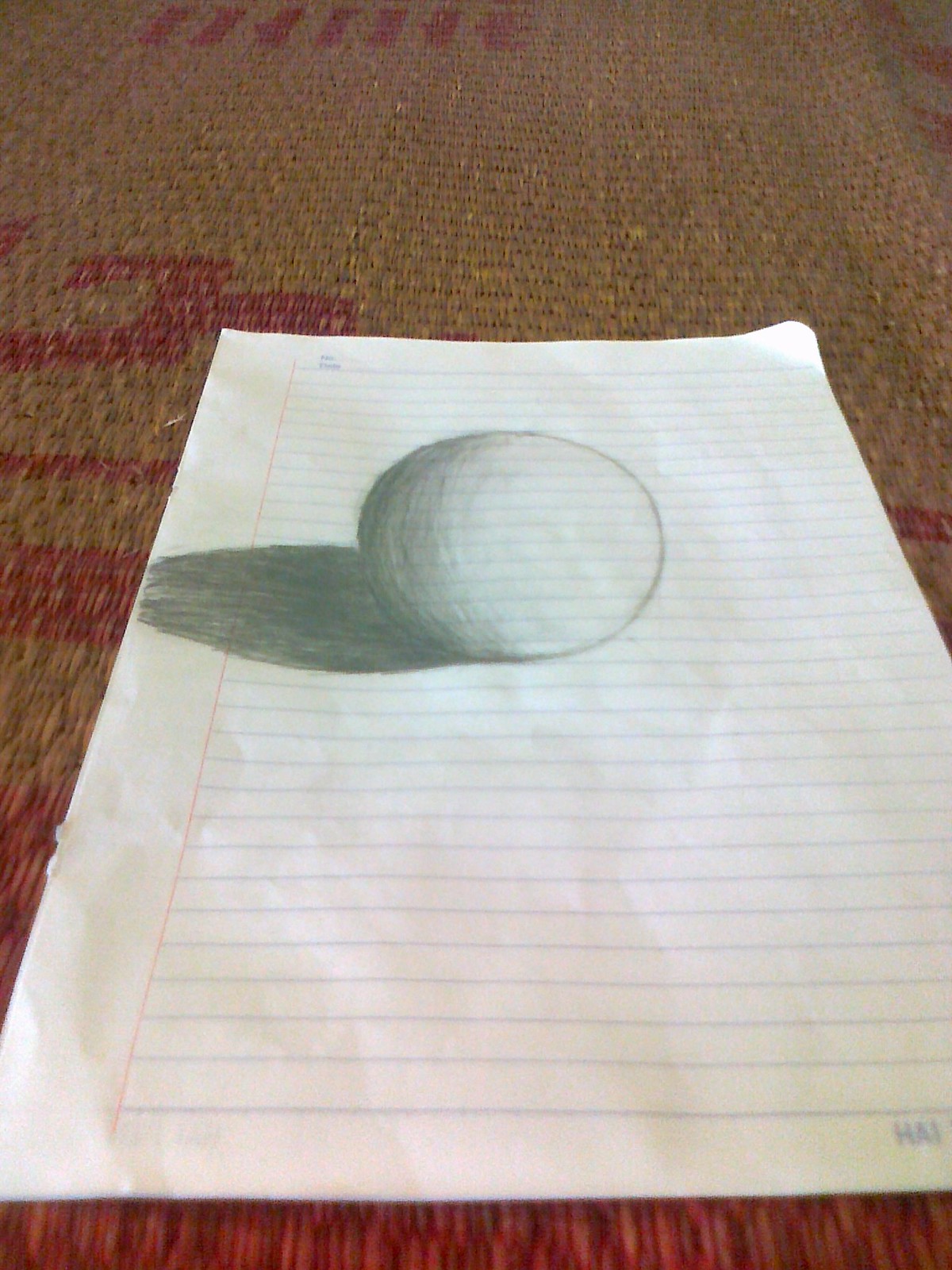The image features a college-ruled lined notepad sheet with blue horizontal lines and a pink vertical margin line on the left. A carefully sketched sphere, occupying nearly half of the page, dominates the center of the paper. The sphere casts a shadow towards the left, adding depth and dimension to the drawing. Underneath the notepad, the surface appears to be a woven basket, with intricate patterns visible. The woven surface is primarily brown, interspersed with patches of red that resemble writing or markings. This combination of elements creates a rich texture and interesting visual contrast in the composition.